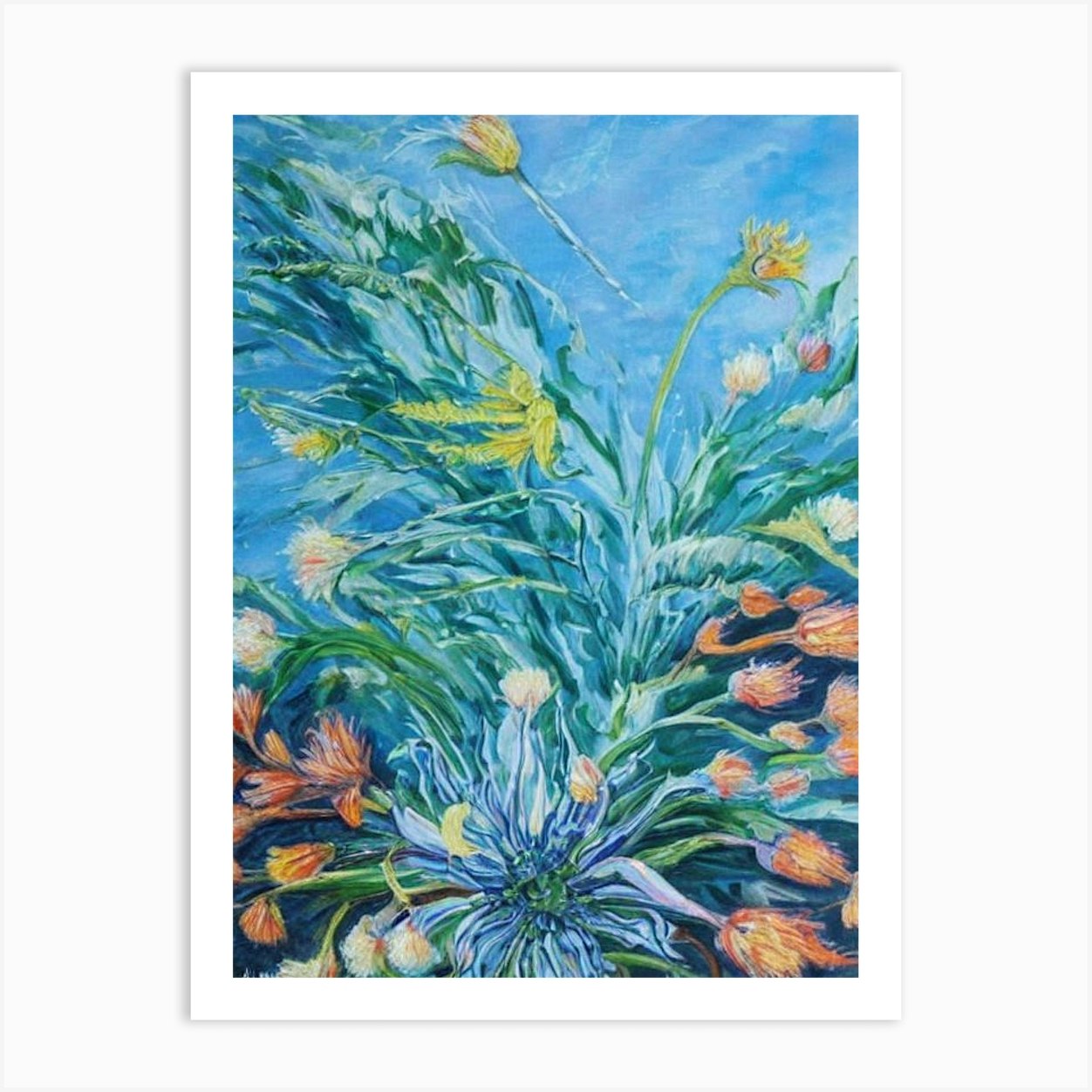The image is a detailed photograph of a painting, possibly created with watercolor or oil pastel, depicting a vibrant underwater or botanical scene. This artwork features a dominant blue petaled flower positioned prominently at the bottom center, surrounded by an array of orange, reddish-yellow, and pink flowers attached to green stems. Long, large green leaves frame the composition, accompanied by slender yellow stalks topped with yellow flowers. The background of the painting is a gradient blue, suggestive of either a sky or underwater environment, and the artwork is bordered by a thin white edge. This entire piece is resting on a separate white surface, casting a slight shadow that differentiates it from the canvas or paper it is on. The combination of these elements creates a cohesive and lively depiction of mixed flora, with rich hues and dynamic arrangements.